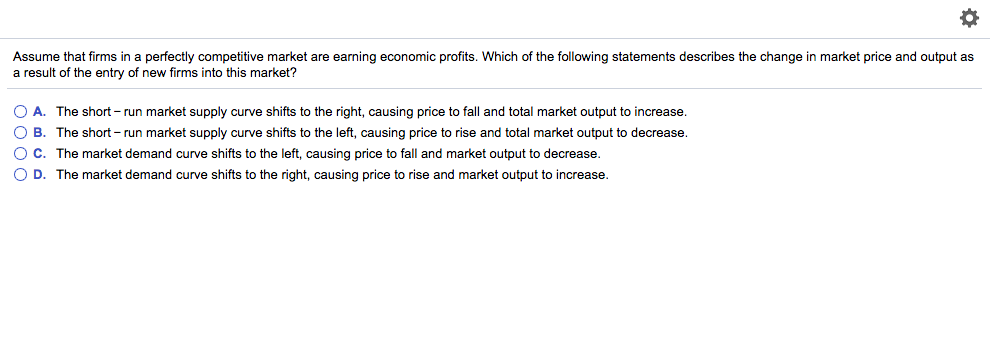On a white background, the upper right corner features a dark grey gear icon. A very light grey horizontal line extends from the left to the right side of the image. In the center, bold black text reads: "Assume that firms in a perfectly competitive market are earning economic profits. Which of the following statements describes the change in market price and output as a result of the entry of new firms into this market?" Following this, there are three blue circles with white interiors, each situated next to a letter (A, B, C, and D), all in blue. 

- Option A reads: "In the short run, the market supply curves shift to the right, causing prices to fall and total market output to increase."
- Option B states: "In the short run, the market supply curves shift to the left, causing prices to rise and total market output to decrease."
- Option C indicates: "The market demand curves shift to the left, causing prices to fall and market output to decrease."
- Option D describes: "The market demand curves shift to the right, causing prices to rise and market output to increase."

The image reflects a multiple-choice question concerning market dynamics in a perfectly competitive environment.